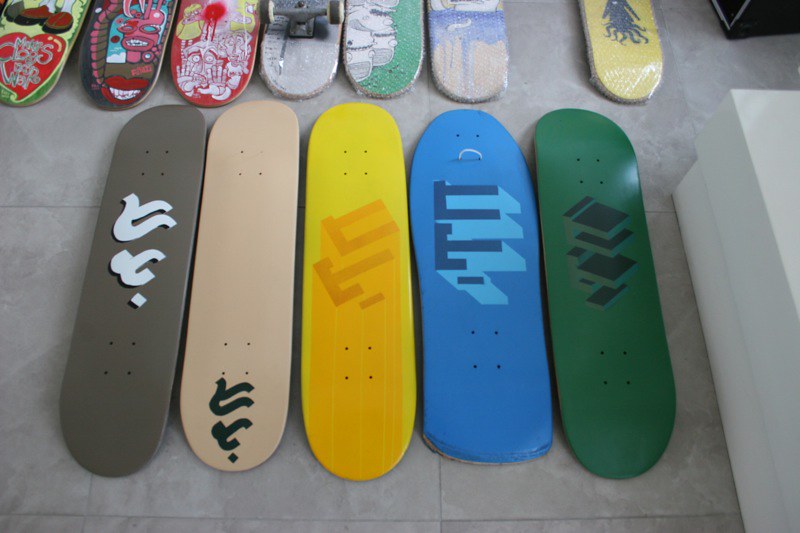This is a horizontally oriented, lower quality color photograph with a cyan tint from natural sunlight. The focus is on five skateboard decks without trucks or wheels, positioned in a row on a light gray linoleum-tiled floor. The skateboards are colored gray, beige, yellow, blue, and green, each adorned with unique symbols or designs. Behind these, several more skateboards are lined up, some wrapped in bubble wrap, and others featuring elaborate, graphic street art. A low white wall extends from the bottom right corner to the top quadrant of the image, where a partially visible box sits. The photograph captures a preparation area for detailing or artistic enhancements on the skateboard decks.